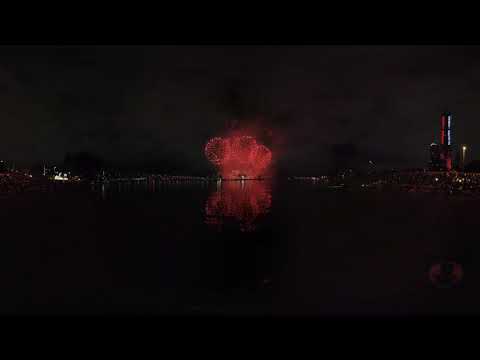The image captures a nighttime scene dominated by darkness, punctuated by a few illuminated points of interest. In the center of the frame, three large, red fireworks burst into spherical patterns. The vibrant red hues of the fireworks contrast starkly against the black sky, and their reflections are visible in the water below, indicating the presence of a waterfront. To the far right, a tall structure resembling a building or a lighthouse, illuminated by red and white lights, stands out against the night. There are also faint, indistinct lights on the far left side of the image, suggesting distant civilization. Overall, the photo presents a serene yet dramatic view of a fireworks display from a considerable distance, with the dark, expansive water in the foreground adding to the sense of vastness and isolation.